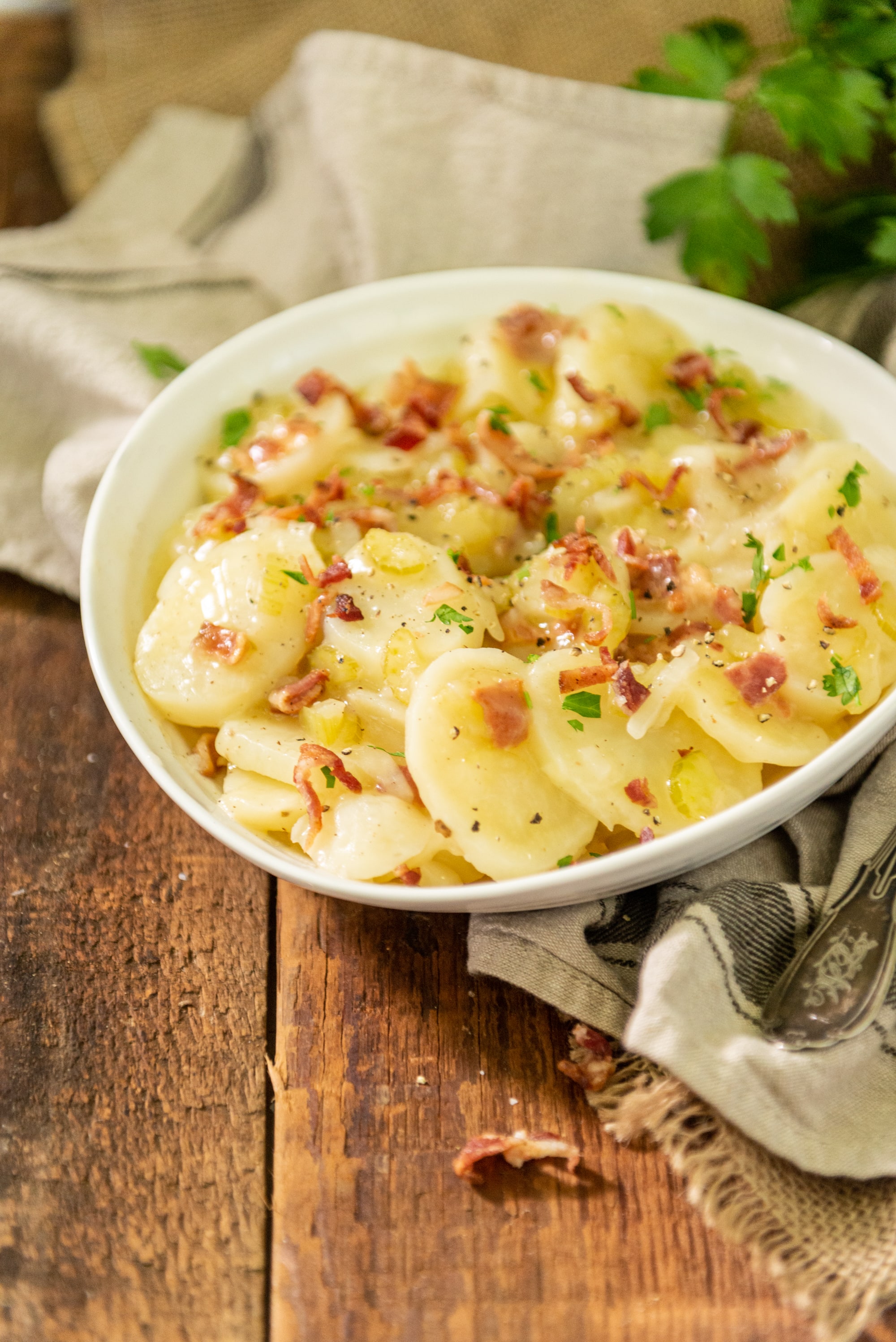A rustic wooden table with weathered slats serves as the backdrop for a culinary presentation. At the center of the table rests a round, white bowl with a partial handle visible on the left side. The bowl showcases a hearty dish of sliced potatoes, generously garnished with crispy bacon bits and finely chopped green parsley. The bowl sits atop an off-white cloth, subtly adorned with brown markings, which peeks out from underneath, giving the arrangement a charming, tucked-in appearance. A vibrant sprig of parsley adds a fresh touch to the composition, positioned delicately in the upper right corner. The entire scene exudes a cozy, inviting atmosphere, highlighting the rustic charm of the setting.